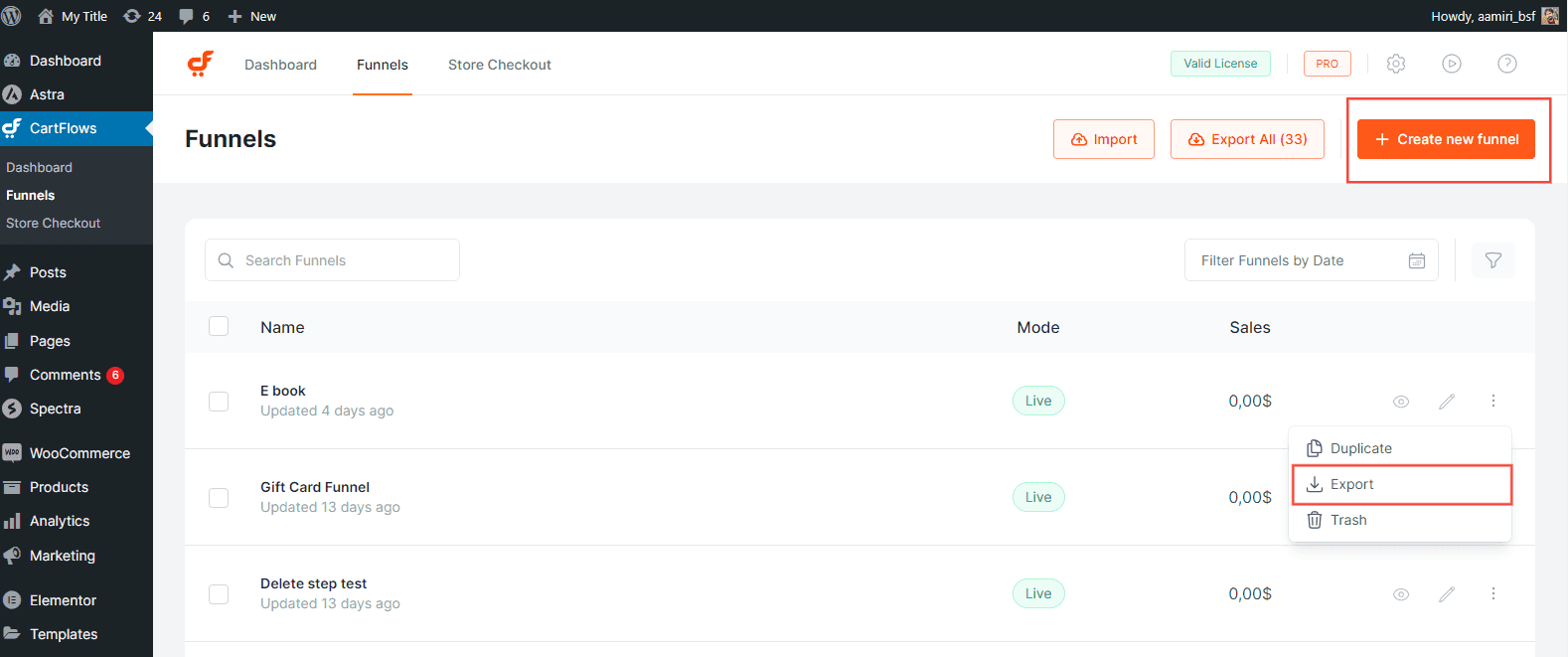Screenshot of a web page featuring a complex interface with multiple navigation elements and an actionable dashboard. On the left-hand side, a black navigation bar displays various categories in white text, including "Dashboard," "Astra," "CartFlows," "Funnels," and "Store Checkout," with "CartFlows" highlighted in blue, indicating selection.

The main content area to the right of the navigation bar is predominantly white. At the top, the CartFlows icon, a red emblem labeled "CF" with small feet underneath, is prominently displayed alongside primary navigation choices: "Dashboard," "Funnels" (outlined in orange and selected), and "Store Checkout." The top right corner features additional icons, followed by the title "Funnels" in bold black text.

On the right-hand side, three interactive buttons appear as pill-shaped bars with orange text: "Import," "Export," and "Create New Funnel." The "Create New Funnel" button is actively selected, demarcated by an orange box housing white text. 

Directly below, a smaller section contains a search bar with filtering options labeled "Filter Funnels by Date," accompanied by a calendar icon for date-based filtering. This section also includes subcategories titled "Name," "Mode," and "Sales."

The interface lists several funnel categories: "E-book," "Gift Card Funnel," and "Delete Step Test," with "Gift Card Funnel" being selected. To the right, options such as "Duplicate," "Export," and "Trash," each paired with specific icons, are presented for the selected funnel. The "Export" option, signified by a down arrow and surrounded by an orange box, is currently chosen.